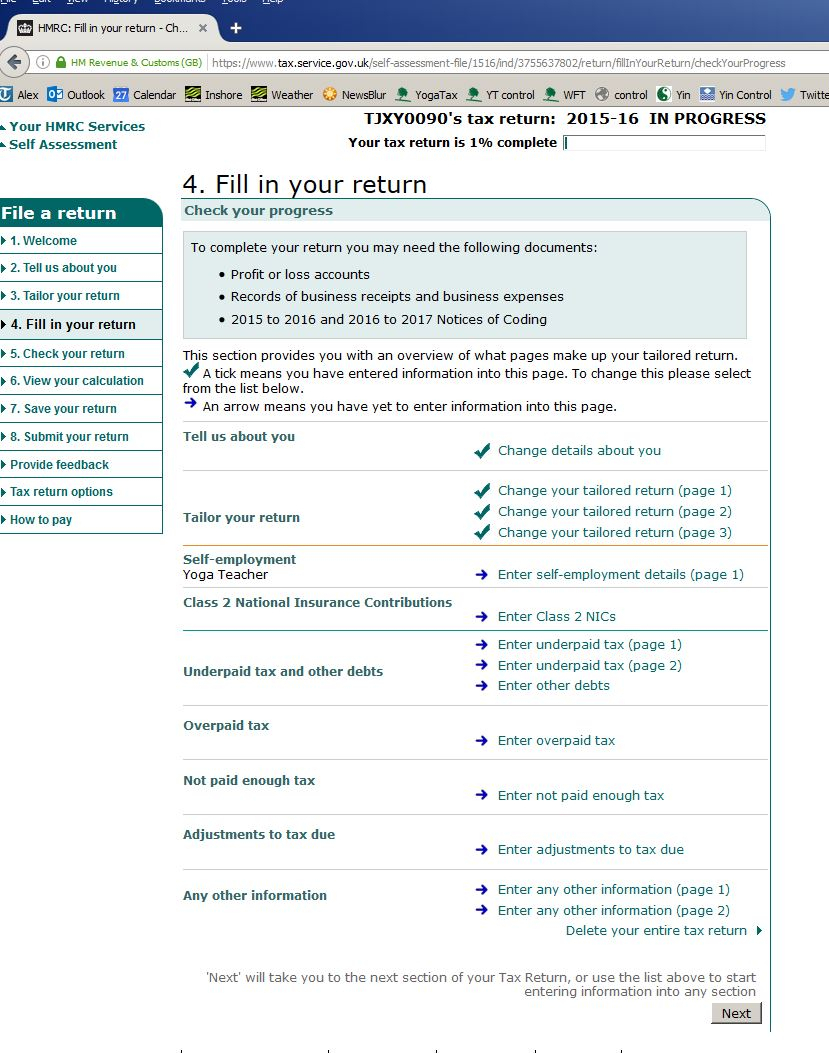The image features a screenshot of an old web browser with a visible tab labeled "HMRC" in capital letters, accompanied by a black logo. The tab appears gray, and there are elements indicating the user's status on the HMRC website. 

At the top left, there's a back arrow and a search bar. The search bar displays "HM Revenue and Customs," suggesting the user is on the official HMRC site. Below the tab area, the gray bookmarks bar lists several bookmarks: "Alex," "Outlook," "Calendar," "Irish Shore Weather," "News Blur," "Yoga Tax," "YT Control," "WFT Control," "YIN Control," and "Twitter."

The main content of the page has a white background. In the upper left corner, bold black text reads, "Your HMRC Services Self Assessment." To the right, it states, "TJXY0090's tax return 2015 to 16 in progress" with a progress bar indicating the return is 1% complete, displaying a small blue line. Below, a green button on the left labeled "File a Return" is in white text.

A numbered menu lists steps for filing the return:
1. Welcome
2. Tell Us About You
3. Tailor Your Return
4. Fill in Your Return (highlighted in light blue, indicating the current step)
5. Check Your Return
6. View Your Calculation
7. Save Your Return
8. Submit Your Return
9. Provide Feedback
10. Tax Return Options
11. How to Pay

On the right, "Fill in Your Return" is highlighted in a light blue bar. Below, a light blue square contains black text: "Check Your Progress. Complete your return. You may need the following documents: Profit or Loss Accounts, Records of Business Receipts and Business Expenses for 2015-2016 and 2016-2017." 

Following this, further instructions provide an overview of the return pages. A blue checkmark indicates completed pages, while a blue arrow signifies incomplete pages. The sections with respective statuses are:

- Tell Us About You: Completed 
- Tailor Your Return: Three completed pages
- Self-Employment, Yoga Teacher: Incomplete 
- Enter Employment Details, Page 1: Incomplete 
- Class 2 National Insurance Contributions: Incomplete 
- Enter Class 2 NICS: Incomplete 
- Underpaid Tax and Other Debts: Incomplete 
  - Enter Unpaid Taxes, Page 1: Incomplete 
  - Enter Unpaid Underpaid Tax, Page 2: Incomplete 
  - Enter Other Debts: Incomplete 
- Overpaid Tax: Incomplete 
- Enter Overpaid Tax: Incomplete 
- Not Paid Enough Tax: Incomplete 
- Enter Not Paid Enough Tax: Incomplete 
- Adjustments To Tax-Due: Incomplete 
- Enter Adjustments To Tax-Due: Incomplete 
- Enter Any Other Information:
  - Page 1: Incomplete 
  - Page 2: Incomplete 

A deletable option "Delete Your Entire Tax Return" is also mentioned. At the bottom of the page, it states, "Next we will take you to the next section of your tax return or use the list above to start entering your information into any section," followed by a gray button labeled "Next" in black text.